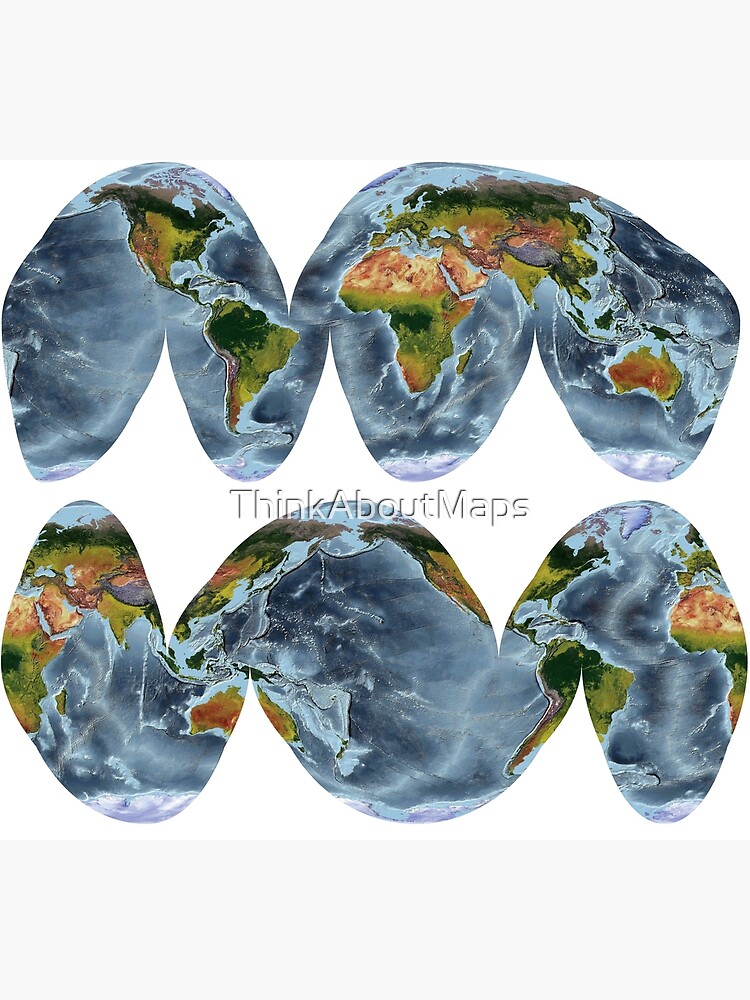The image depicts a stylized map of the Earth, represented within a bubble letter "M" shape that end with an additional segment, reminiscent of a worm-like structure. The map is arranged in a split, wavy pattern which reveals both hemispheres in a peeled, continuous layout, with the top and bottom sections mirroring each other. The background is a light blue, much lighter than natural water bodies, creating a distinctive contrast. The continents are displayed with a mix of greens and yellows, with Africa notably featuring brown areas indicative of desert regions. 

At the top of the structure, you can distinguish North and South America, Africa, and Europe, while Australia is visible in the upper section. The oceans are depicted in a blend of blues and grays, occasionally interspersed with white highlights and clusters of islands, which gives the impression of an x-ray design layered over the map.

The bottom section showcases similar geographic elements, suggesting alternate views of the same countries from different angles, with color schemes consistent with the top—green, dark green, yellow, and brown for land, and blues and grays for water. At the center of this intriguing composition, the phrase "Think About Maps" prominently captures attention, emphasizing the unique and creative representation of the world’s geography.